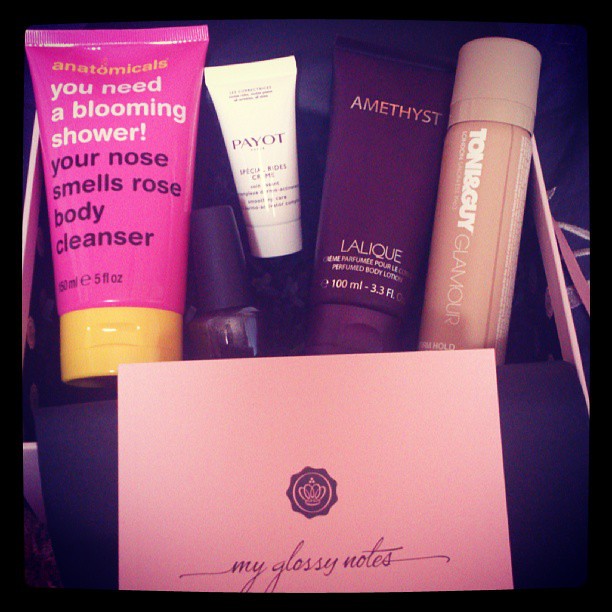This is a full-color photograph of a gift box containing five beauty and self-care products, all positioned neatly inside. The box itself is black, accented with a pink envelope at the front, sealed with a crown and inscribed in purple cursive with "My Glossy Notes." The borders of the photo are thicker on the sides compared to the top and bottom.

The first item, prominently displayed on the left side, is a pink tube with a yellow lid labeled "Anatomicals You Need a Blooming Shower Your Nose Smells Rose Body Cleanser." To its right, a smaller white tube features the brand name "Payot," though the exact product name is hard to discern due to small print. Following that is a dark gray bottle, presumed to be nail polish, its identity partially obscured as the writing is not visible. The fourth item is a black tube labeled in white letters with "Amethyst La Leak" and the volume of 100 milliliters. Finally, the fifth product is a beige container marked "Tony and Guy Glamour." The presentation in the box suggests it is curated as a self-care or beauty set, despite the photograph not being of the highest quality.